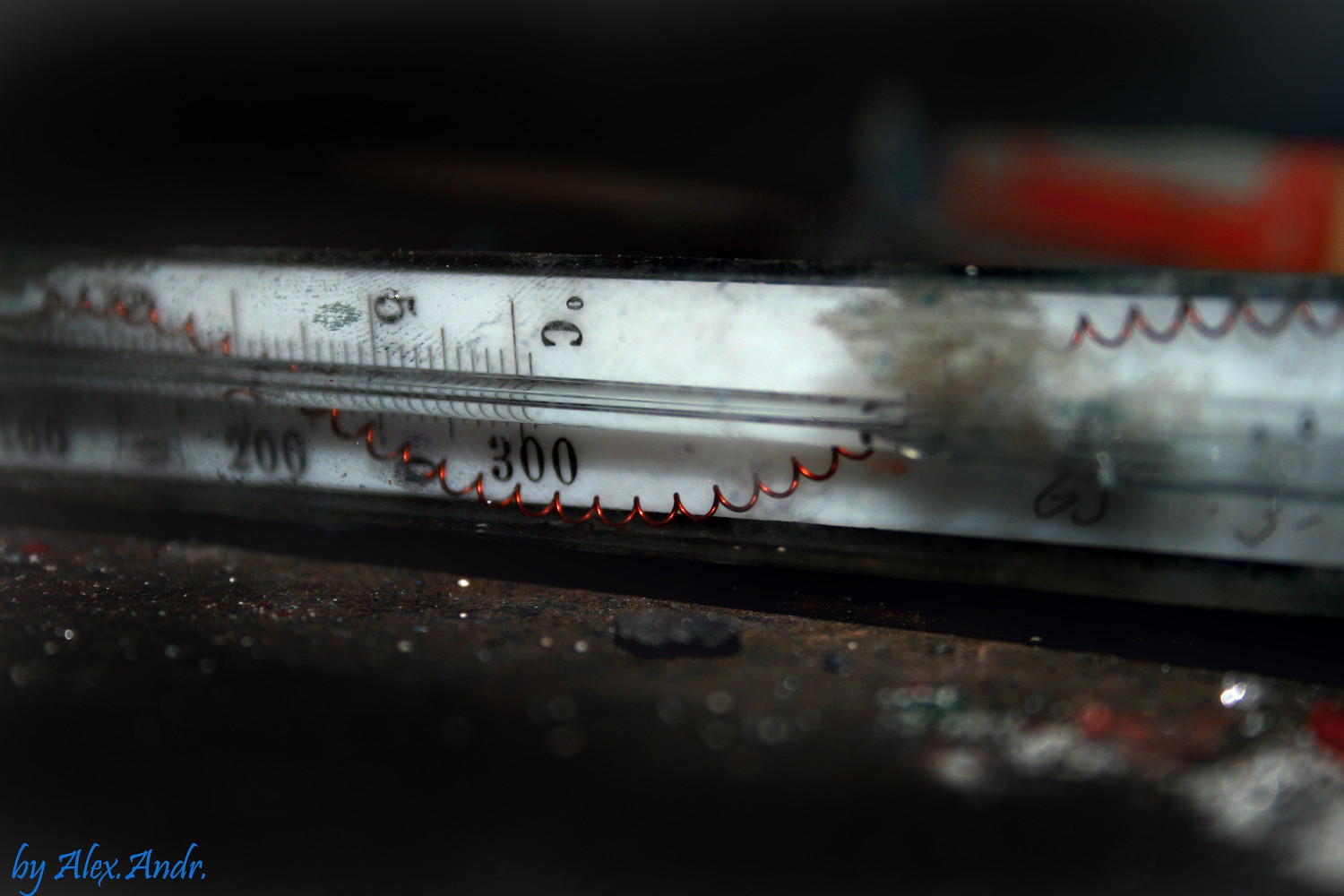A close-up photograph captures a weathered thermometer lying on its side. The thermometer's face is protected by a broken glass case, revealing a white background with black numbers and letters indicating Celsius readings. Notably, the glass column encloses the mercury, which is crucial for its temperature gauging function. 

In the bottom left corner of the image, the phrase "by Alex.andr" is stylishly inscribed in a fancy blue font. The surface of the thermometer shows signs of adhesive residue, marked by a dirty tape smudge and scattered fingerprints. The casing of the thermometer seems to be made of either a thin black metal or plastic material.

Drawing the eye further, a slender red wire coil reminiscent of spiral notebook binding drapes around the thermometer. This shiny red wire extends the length of the visible thermometer, weaving from the top left, behind the mercury column, and exiting to the right.

The thermometer rests on a gritty surface littered with reflective particles, possibly resembling mica or metal shards, adding to the overall aged and dirty appearance of the scene. A blurred, flat pebble lies in the foreground, contributing to the photograph’s textured and cluttered aesthetic.